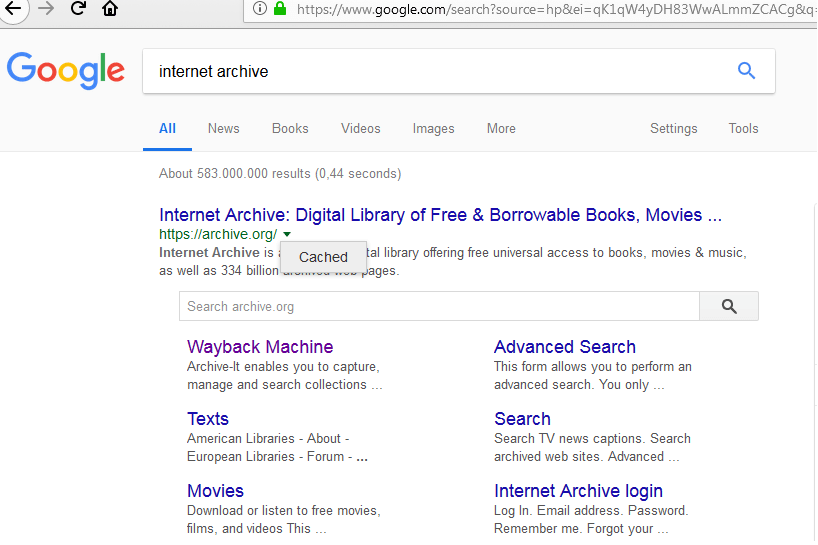The website interface shown in the image is Google Search. In the top left corner of the browser are navigation buttons including left and right arrows, a refresh icon, and a home button. Adjacent to these is a secure connection symbol indicated by a green lock, followed by the URL "https://www.google.com/search?source=hp&ei=QK1QNW41DHA3WWALMMNCCACGNQ". The prominently displayed Google logo is colored with blue for "G", red for "o", yellow for "o", blue for "g", green for "l", and red for "e". 

Below this, the search bar appears containing the inner archive search criteria. The menu options below the search bar are categorized as "All", "Books", "Videos", "Images", "More", "Settings", and "Tools". The search yields approximately 583 million results in just 0.44 seconds. 

The snippet showcases "Inner Archive", described as a digital library offering free access to books, movies, and music. The URL associated with this library is "https://archive.org". This platform, known for the Wayback Machine and other advanced search tools, facilitates users in capturing, managing, and searching collections. The highlighted results emphasize that users can search TV news, collections, and download or listen to free media like movies, films, and images from the archive.